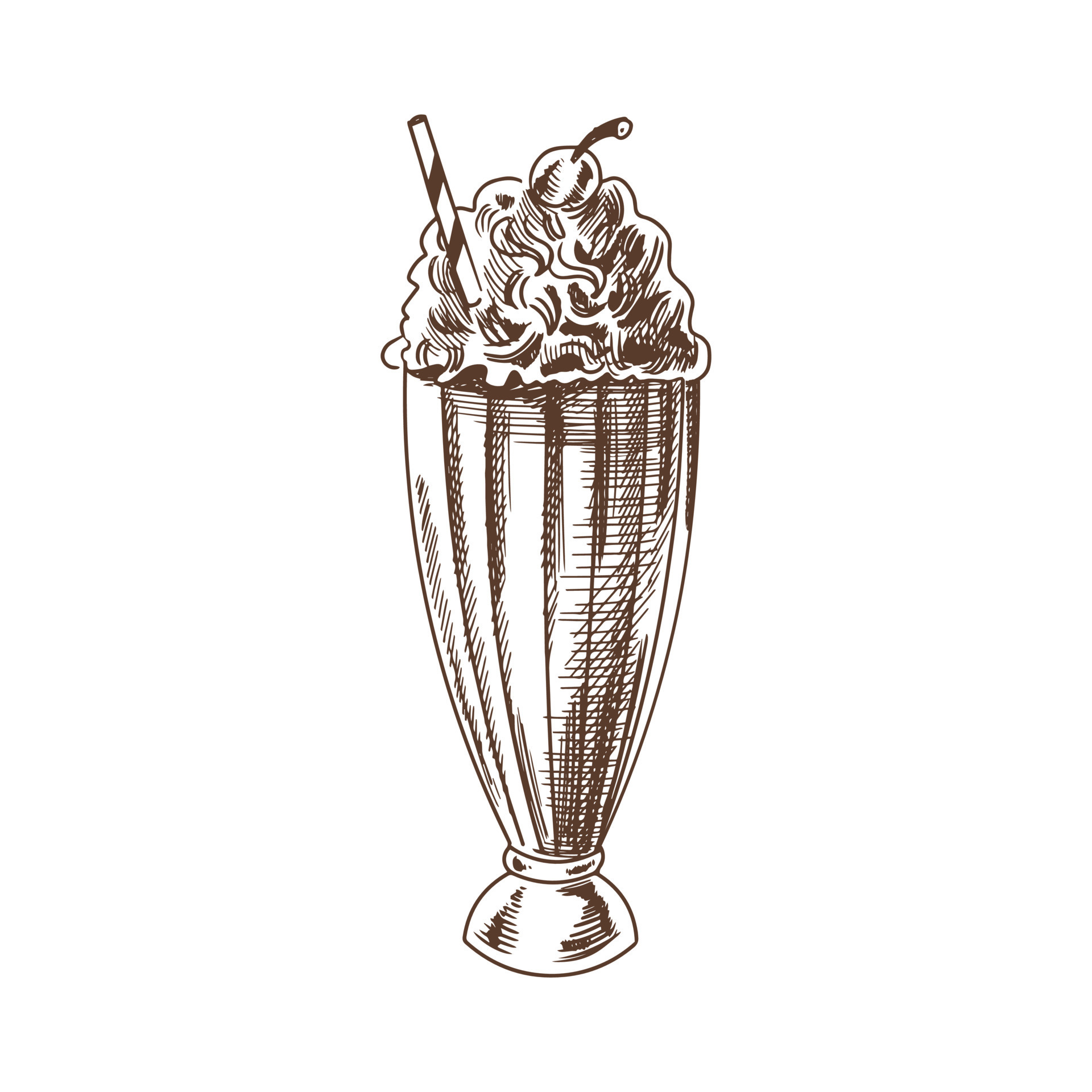The image is a detailed, stylized black and white drawing of a milkshake in a tall, classically fluted glass with a small round base. The flutes run vertically up and down the body of the glass, giving it a distinctive vintage soda shop appearance. Shading with thick pencil lines on the right and top, along with thinner lines on the left, suggests depth and shadows. The milkshake is topped with a generous pile of swirly whipped cream, characterized by pencil-scalloped edges and detailed cross-hatching. Garnishing the top is a maraschino cherry with a stem pointing to the right and a striped straw inserted on the left side. The image is rendered on a transparent background, giving it a clip-art-like quality, but in a larger, more intricate format.